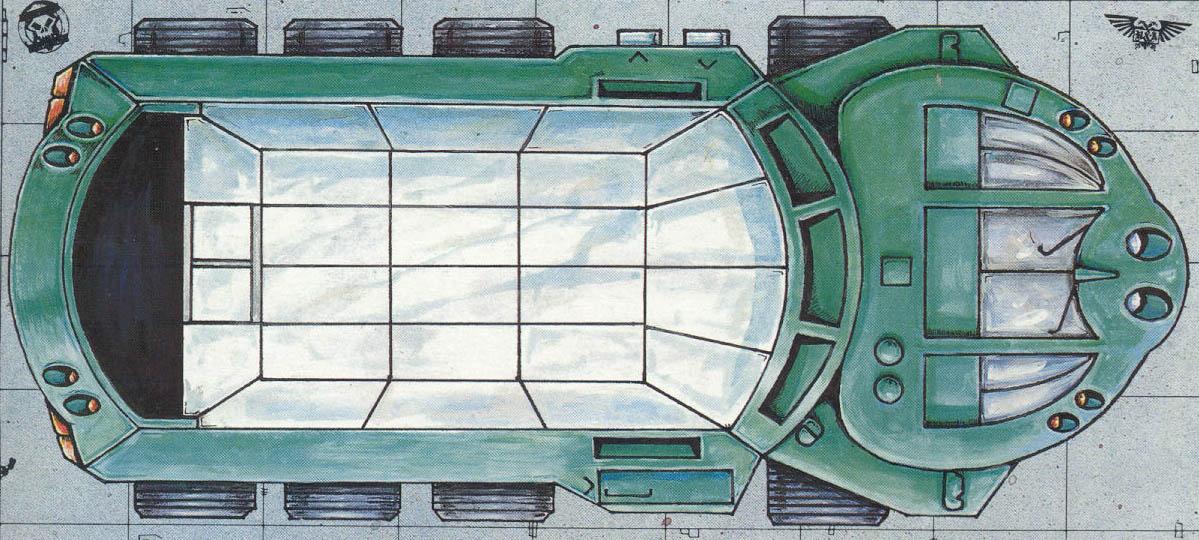This hand-drawn illustration, viewed from above, depicts a futuristic truck with a greenish cab that has multiple windows, headlights, and side lights. The vehicle's cargo area, which resembles a dump truck, features a whitish-grayish interior with a subtle blue hue, possibly due to reflections. The truck has a total of eight wheels, three sets of two smaller wheels at the back and two larger wheels near the front. The entire scene is laid over a tiled cement background that is light gray with a slight green tint. In the top corners of the image, there are two logos: a skull-like emblem on the left and a bird-like symbol on the right. The truck's design includes orange taillights and evokes a slightly cartoony artistic style, suggesting it might be drawn by a non-professional artist, possibly a teenager. The overall impression is of a detailed and imaginative, though somewhat ambiguous, landscape-oriented drawing of a vehicle.